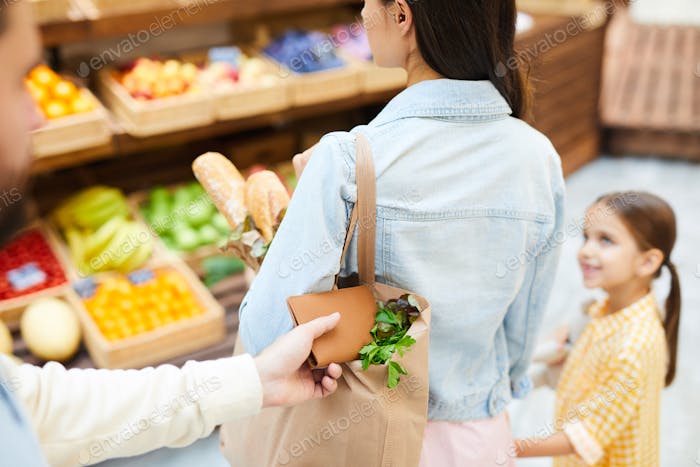In a somewhat blurred photograph taken in a grocery store, a woman with long, straight, dark brown hair, dressed in a collared denim shirt, stands in the middle of the image. Her head is slightly cut off at the top of the frame. She carries a light beige shoulder bag, slung over her left shoulder, which contains two loaves of French bread and some leafy produce sticking out. Unbeknownst to her, a person with a long white sleeve is seen in the lower left corner, reaching into her bag to pull out a brown wallet, nearly fully extracted. To her right stands a young girl, approximately six or seven years old, with a long brown ponytail and a checkered pink and white short-sleeve shirt. The girl is looking up at the woman with a smile on her face. Around them, particularly on the left side of the image, are baskets filled with various produce items like bananas, oranges, and green apples. In the image's upper right corner, some blurred wood slats are visible.